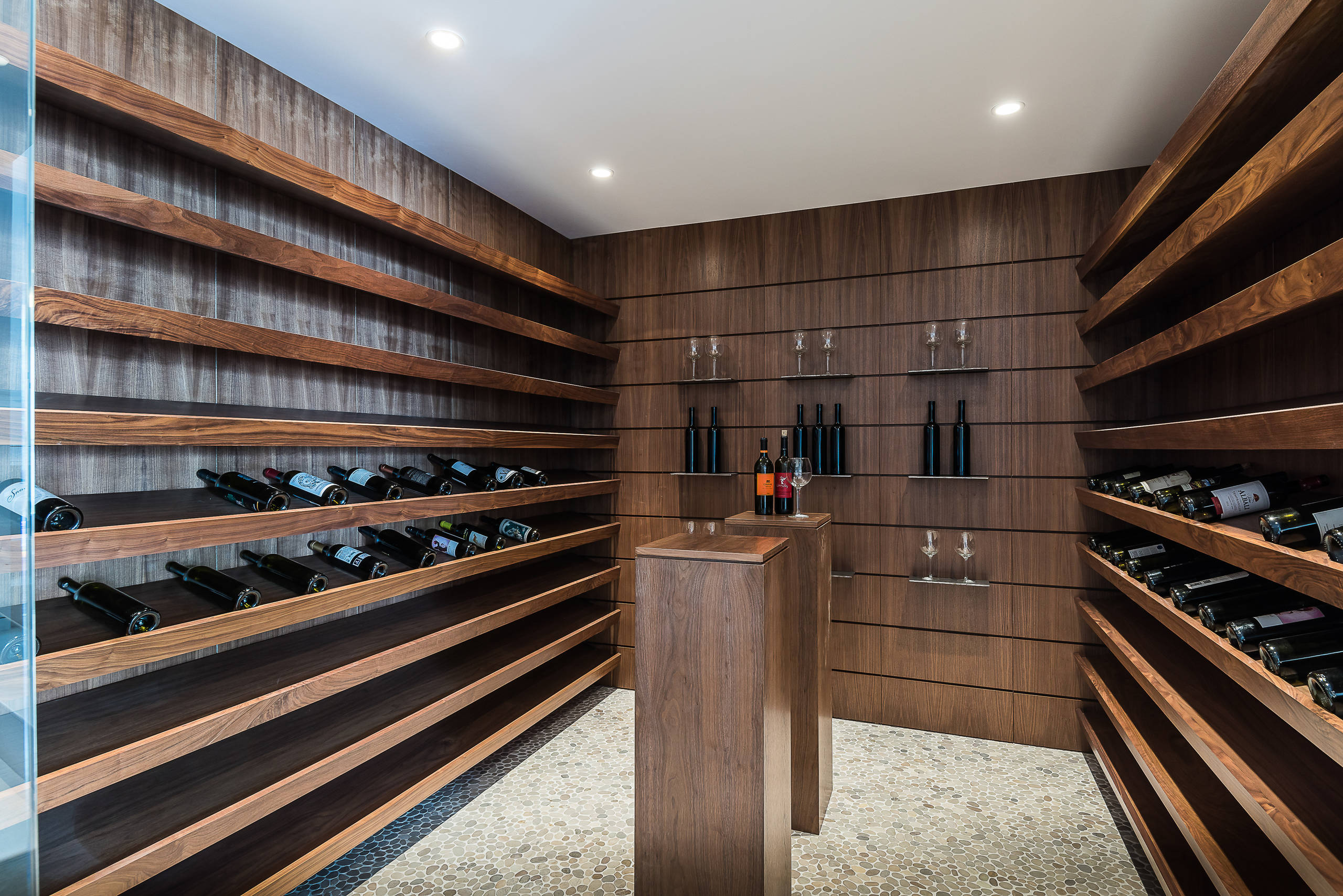This high-quality color photo captures the interior of a sophisticated wine cellar with deep dark wooden panels. The cellar features long, tilted shelves lining both the left and right walls, each wall having nine shelves, two of which on each side hold evenly spaced, dark-colored wine bottles. The center of the wine cellar showcases two four-foot-tall wooden podiums, one of which displays two bottles of wine and a wine glass. The far wall of the cellar serves as a display area with nine individual shelves arranged in three rows. The top and bottom rows each hold two wine goblets on every shelf. The middle row presents a symmetrical arrangement, with two wine bottles on the left shelf, three in the center, and two on the right, all without labels. The floor is made of elegant marble, adding to the overall grandeur of the space.